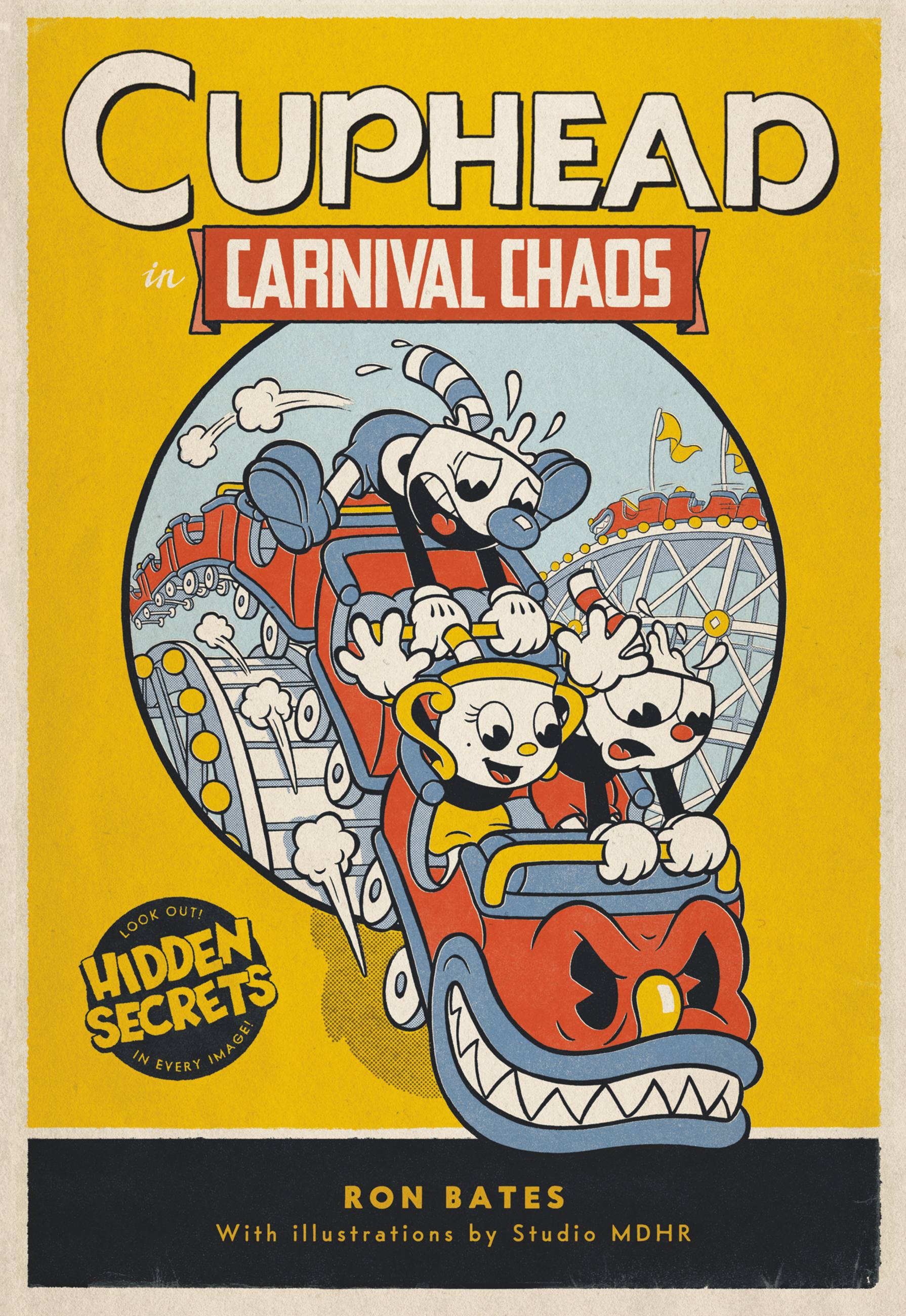The cover page, reminiscent of a vintage comic book, showcases the vibrant scene of "Cuphead in Carnival Chaos," a children's book titled in large white font on a yellow background with a cream-colored outer border. The title is prominently featured, with "Cuphead" in large white letters and "Carnival Chaos" situated within a brown ribbon design. Below the title, a thrilling carnival ride bursts through a circular portal-like design, carrying animated characters who resemble classic Mickey Mouse-style figures, with white gloved hands, stick-like black arms, and expressive faces. The coaster cart itself is alive with an evil-looking face, complete with scary eyes and sharp teeth, adding a sense of danger to the ride. The scene is enlivened with colorful flags and twisting ride tracks, suggesting high-speed excitement. In the bottom left corner, a black logo warns, "Look out, hidden secrets in every image," printed in yellow. The bottom strip, also black, credits Ron Bates as the author, with illustrations by Studio MDHR, tying together the engaging and detailed cover design.